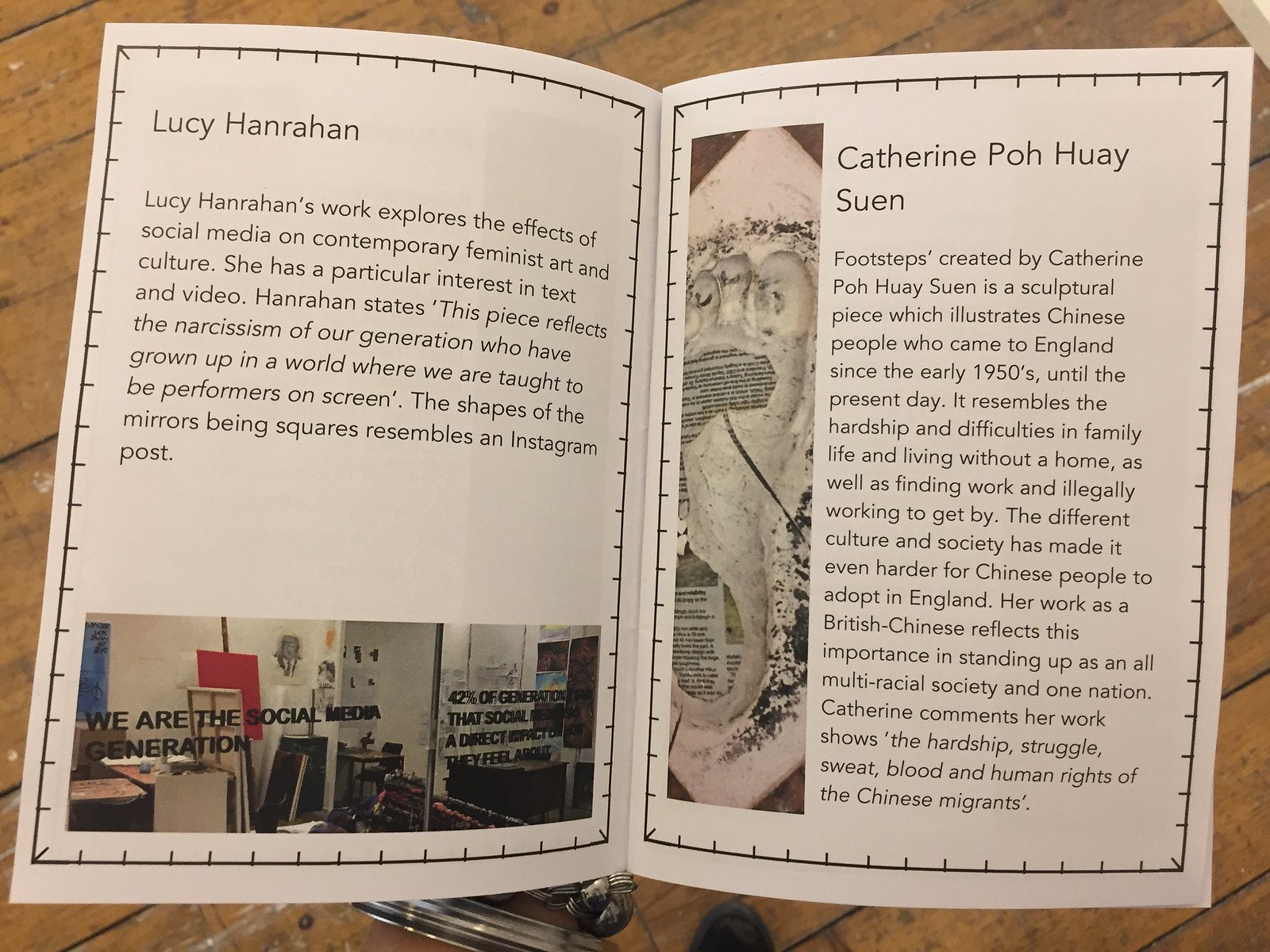This is a photograph of a brochure for an art exhibit, laid open on a wooden table. The brochure features two pages, each dedicated to a different artist. Both pages have a black border resembling staples around the edges. 

On the left page, the title reads "Lucy Hanrahan." Below the title, there is a paragraph describing Hanrahan's work, which explores the effects of social media on contemporary feminist art and culture. She has a particular interest in text and video. A quote from Hanrahan states, "This piece reflects the narcissism of our generation who have grown up in a world where we are taught to be performers on screen." Beneath this text is a photograph that appears to be taken through a window of an art studio, showing paint easels and assorted artworks. The window has the words "we are the social media generation" and some additional blurry text about the impact of social media.

On the right page, titled "Catherine Po-Wai Swen," there are two paragraphs providing a biography of Swen. To the left of the text is an image of what appears to be a sculpture of a foot. The detailed layout suggests that the brochure showcases biographies and samples of work from different artists.